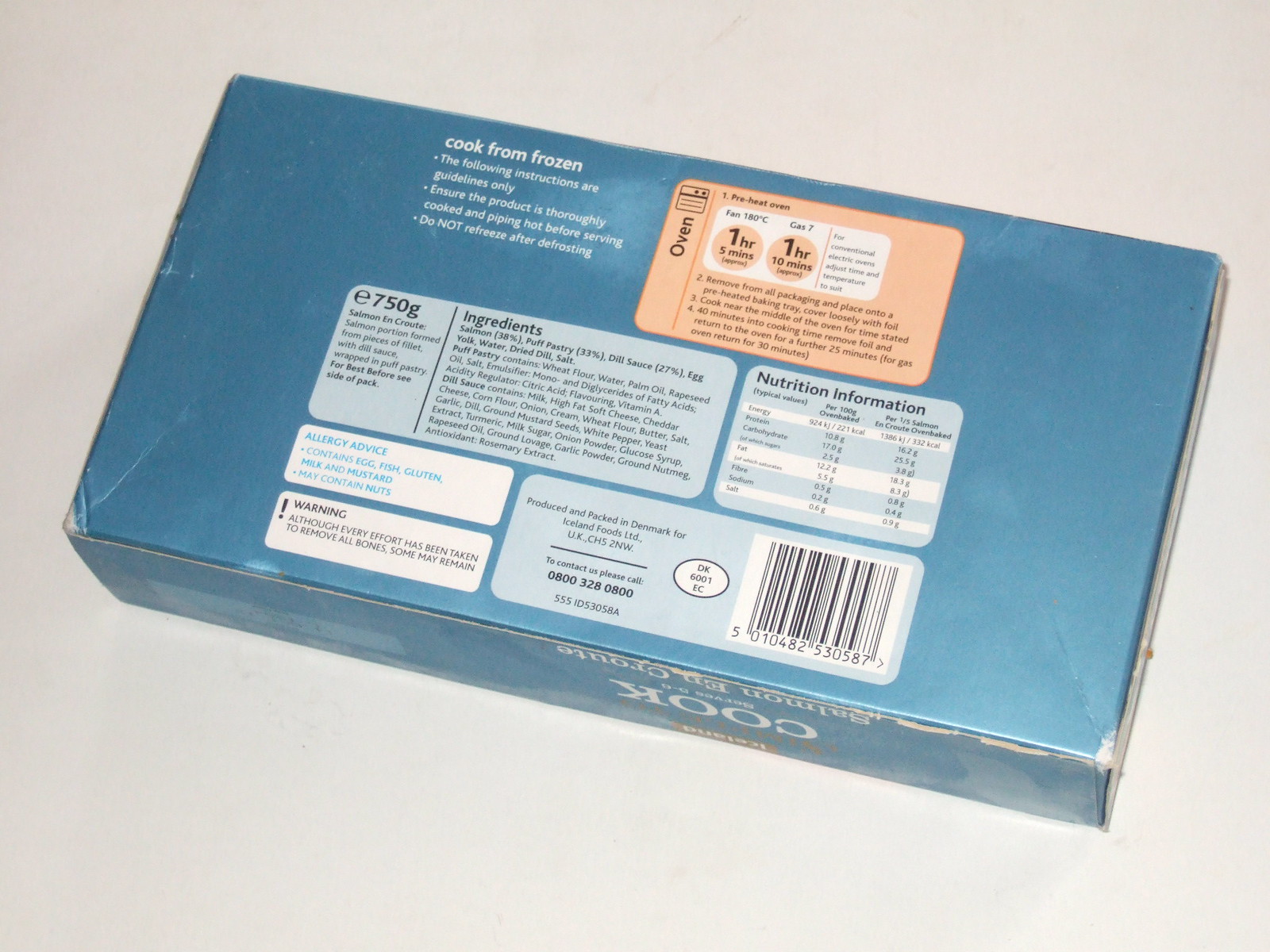In this photograph, the backside of a food package is prominently displayed, oriented somewhat upside down but still legible. At the very bottom of the packaging, the words "Cook" and "Salmon en Croûte" are visible. The focus is primarily on the back of the package, where detailed cooking instructions are provided.

In the top left corner, a notice reads, "Cook from frozen. The following instructions are guidelines only. Ensure the product is thoroughly cooked and piping hot before serving. Do not refreeze after defrosting." To the right of this notice, there is an orange rectangular box labeled "Oven," which contains the cooking instructions. 

Step-by-step instructions are detailed as follows:
1. Preheat the oven to fan 180 degrees Celsius or gas mark 7. Two circles underneath indicate the cooking duration, one hour and five minutes, and one hour and ten minutes.
2. Remove the product from all packaging and place it onto a preheated baking tray, covering it loosely with foil.
3. Cook near the middle of the oven for the time stated.
4. Forty minutes into the cooking time, remove the foil and return the product to the oven for a further 25 minutes (30 minutes for gas ovens).

Below these instructions, several other sections are visible. One box displays the ingredients list, another provides nutritional information, and there is a section with production details, including the location of production and a barcode. To the left, there is an allergy advice section and a warning to remove all bones before consumption.